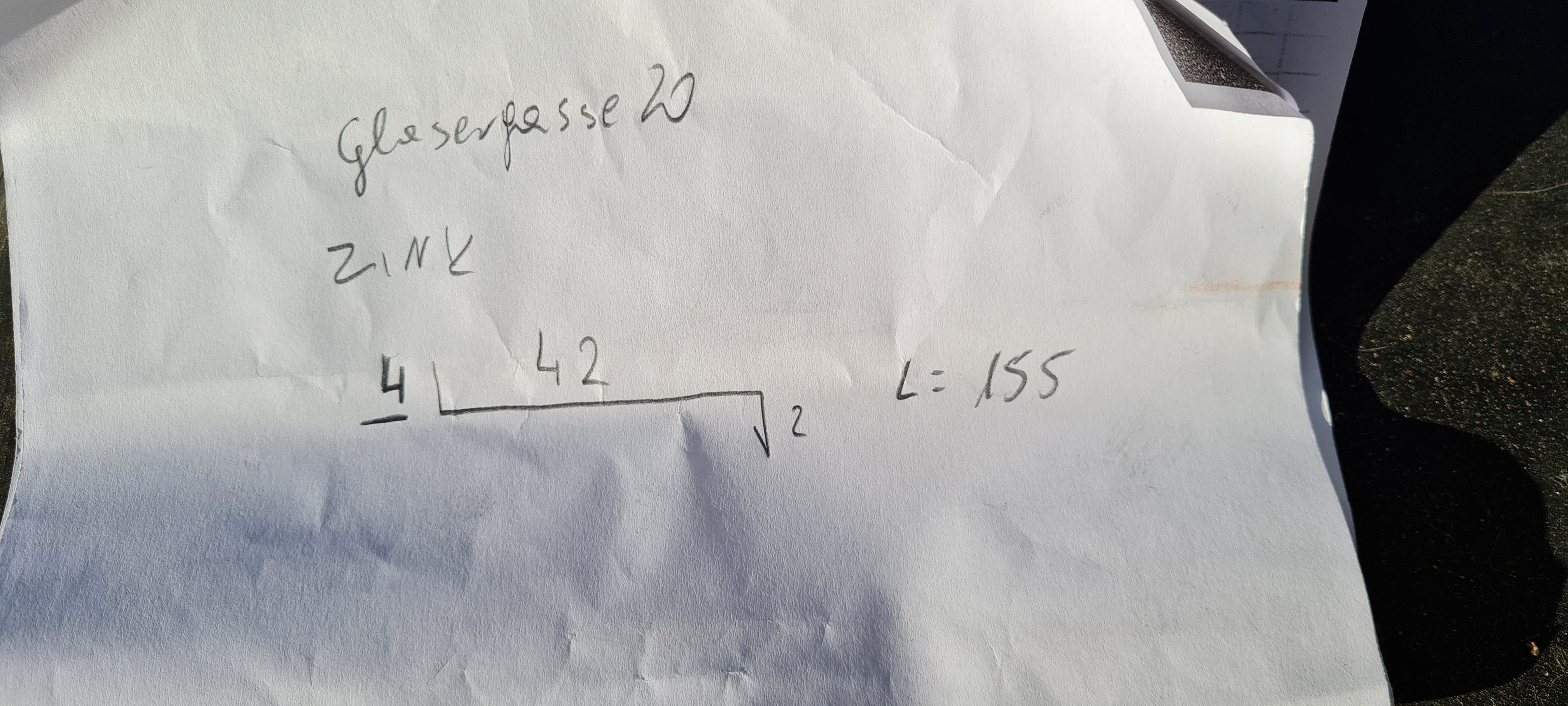The photograph depicts a piece of standard white computer paper resting on a rough black surface, possibly asphalt, indicating an outdoor setting with natural sunlight casting shadows. The paper is positioned amidst a wider-than-average rectangular frame. Behind it, two additional pieces of paper are partially visible, though details are predominantly discernible on the foremost sheet. The paper lies slightly curled at the top right corner, revealing a small black square underneath. 

To the immediate right, a shadow curves elegantly in an oval shape, extending towards the top right of the image. The third paper behind the main one features a hand-drawn graph in pencil, albeit only partially visible.

The primary sheet bears handwritten text and mathematical notations. The text, written in cursive, reads "GlaserPasse20" and directly below that, "ZINY". Additional markings include a mathematical expression with a square root, the number 42, another number 2, and the notation "L=155." 

The contrasting textures of the paper against the rough, scratched surface and the interplay of light and shadow contribute to the image's tactile and dynamic qualities.